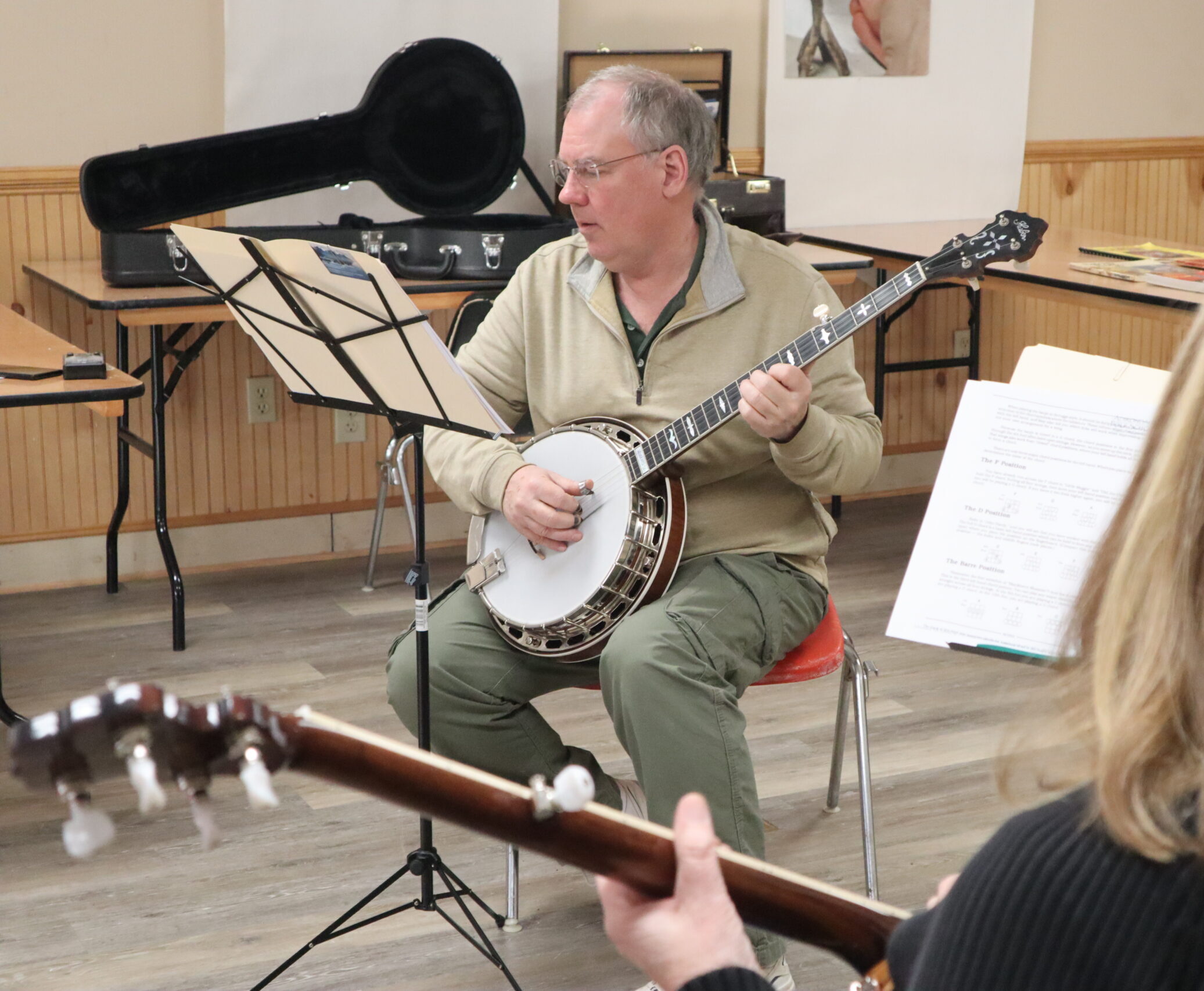In the center of the image, an older man, possibly in his late 50s or early 60s, is seated on an orange chair with metal legs, engrossed in playing a banjo. He has short gray hair and wears glasses, paired with a light-colored sweater and olive green pants. His body faces slightly to the left, but his head is turned more sharply in that direction as he focuses intently on sheet music placed on a black music stand to his left. Behind him, on the left side of the image, stands a table with an open black banjo case, and to his right, another table is present, running perpendicular to the first with a background wall that is light-colored on top and features wood paneling at the bottom. The bottom right corner of the image reveals part of another person’s shoulder-length blonde hair, their blue sweater-clad left shoulder, and a hand grasping the neck of a string instrument, likely another banjo, creating a layered, intimate scene of musical practice. Additional sheets of music on a stand are partially visible to the right of the blonde-haired figure, though the stand itself is obscured.